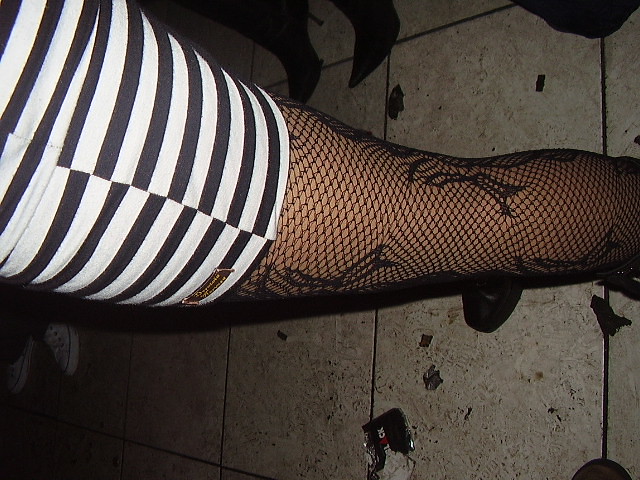This photograph, presented in landscape orientation but captured in portrait, depicts a close-up view of a woman's leg, standing on tiled flagstones with scattered debris, possibly litter or a cigarette pack. The woman is adorned in ornate fishnet stockings embroidered with floral patterns, and she wears a short, above-the-knee skirt or dress characterized by black and white horizontal stripes. Her black shoes stand out against the lightly littered tiles. Also visible are pointy-toed boots of another person standing behind her, suggesting a queue or gathering. The angled perspective, likely taken from behind and to the left of the woman, adds to the intriguing composition of the image.